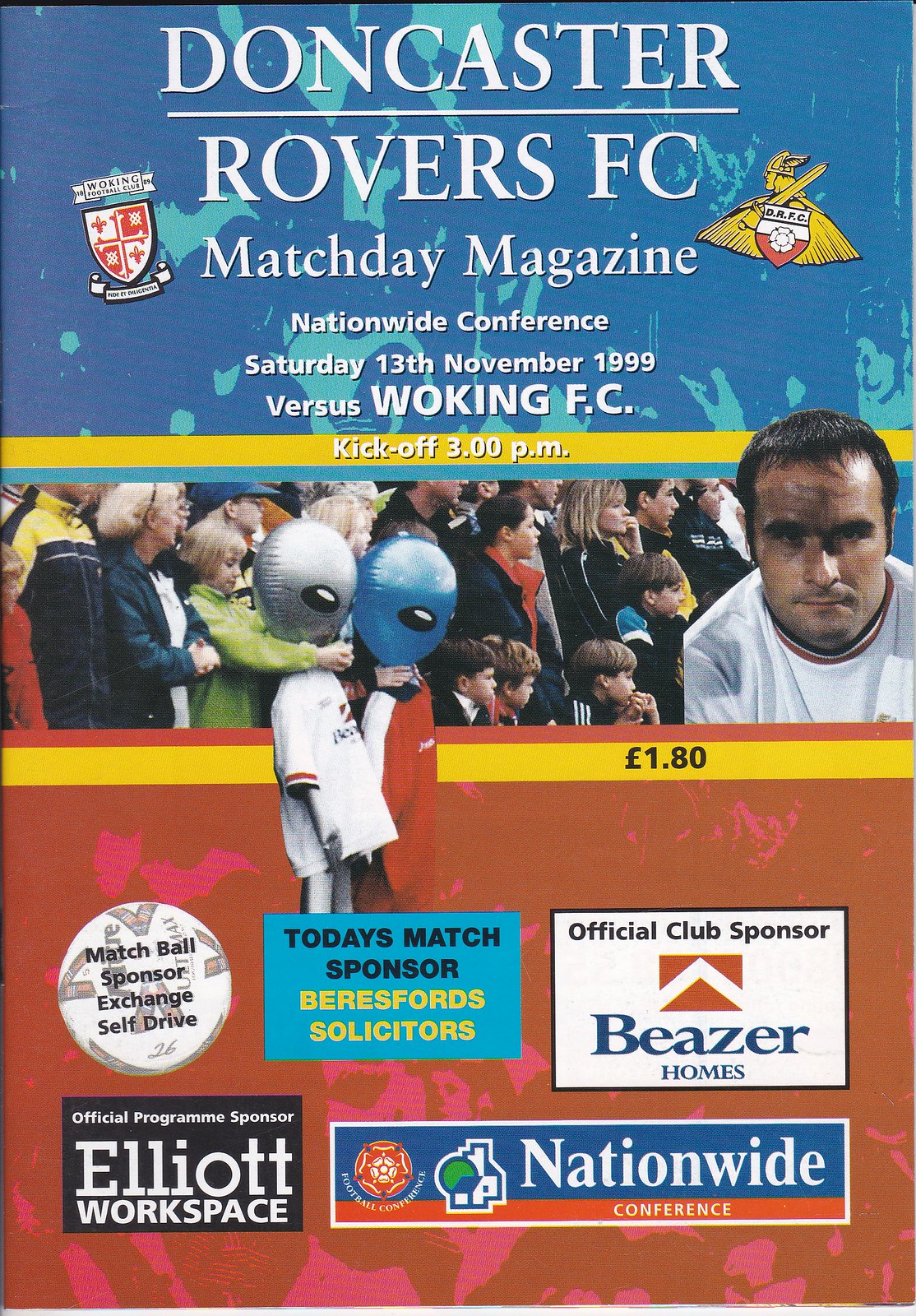The image is a scanned cover of a Doncaster Rovers FC matchday magazine from the Nationwide Conference, detailing the game against Woking FC on Saturday, November 13th, 1999, with a kickoff at 3 p.m. The top part of the cover features a blue background with a slightly lighter blue splatter pattern. The text "Doncaster Rovers FC Match Day Magazine Nationwide Conference Saturday 13th November 1999 Versus Woking FC" is prominently displayed in white, flanked by logos on both sides. Beneath this, a yellow bar with white text announces the kickoff time.

The central image showcases a crowd of fans, including two children holding up aluminum balloons shaped like alien soccer players. Among the crowd is a close-up bust of a soccer player in a white jersey with a red and black collar, gazing directly at the viewer. 

At the bottom of the cover, in a series of colored blocks and text, various sponsors are listed: "L1.80" for the magazine price, "Match Ball Sponsor Exchange Self-Drive," "Today's Match Sponsor Beresford Solicitors," "Official Club Sponsor Beezer Homes," and "Official Program Sponsor Elliott Workspace," all on a red background.